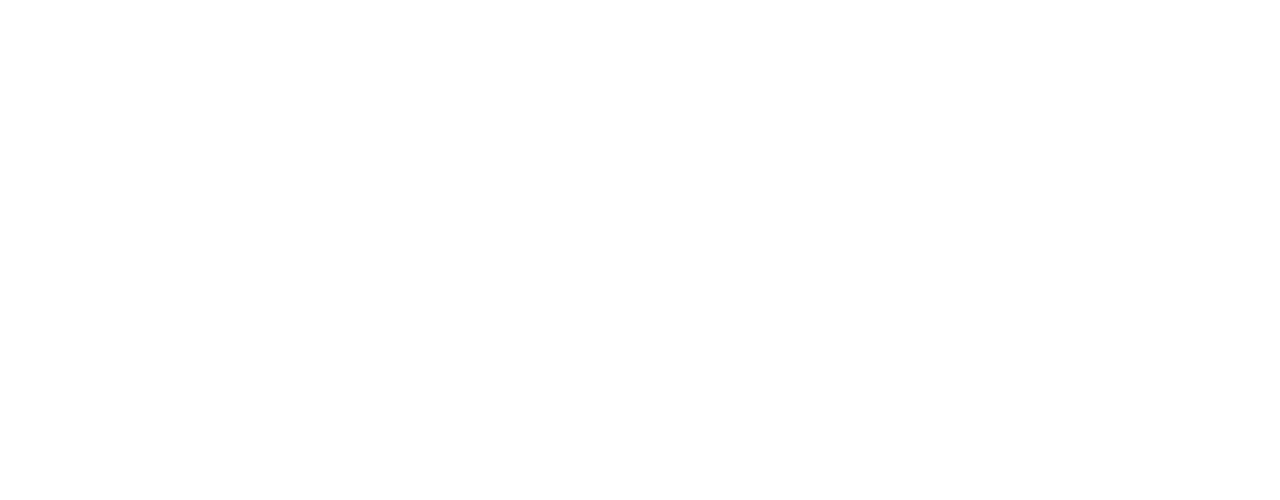The image appears to be a completely blank, white screen with no visible content or edges. Multiple attempts to reload or refresh the screen did not resolve the issue, indicating it is likely a technical error rather than a processing delay. This all-white backdrop suggests that no photograph or image has been loaded or displayed. Users have consistently noted the absence of any visual elements, and this lack of content has been unusual compared to previous surveys where images typically appear without issue.